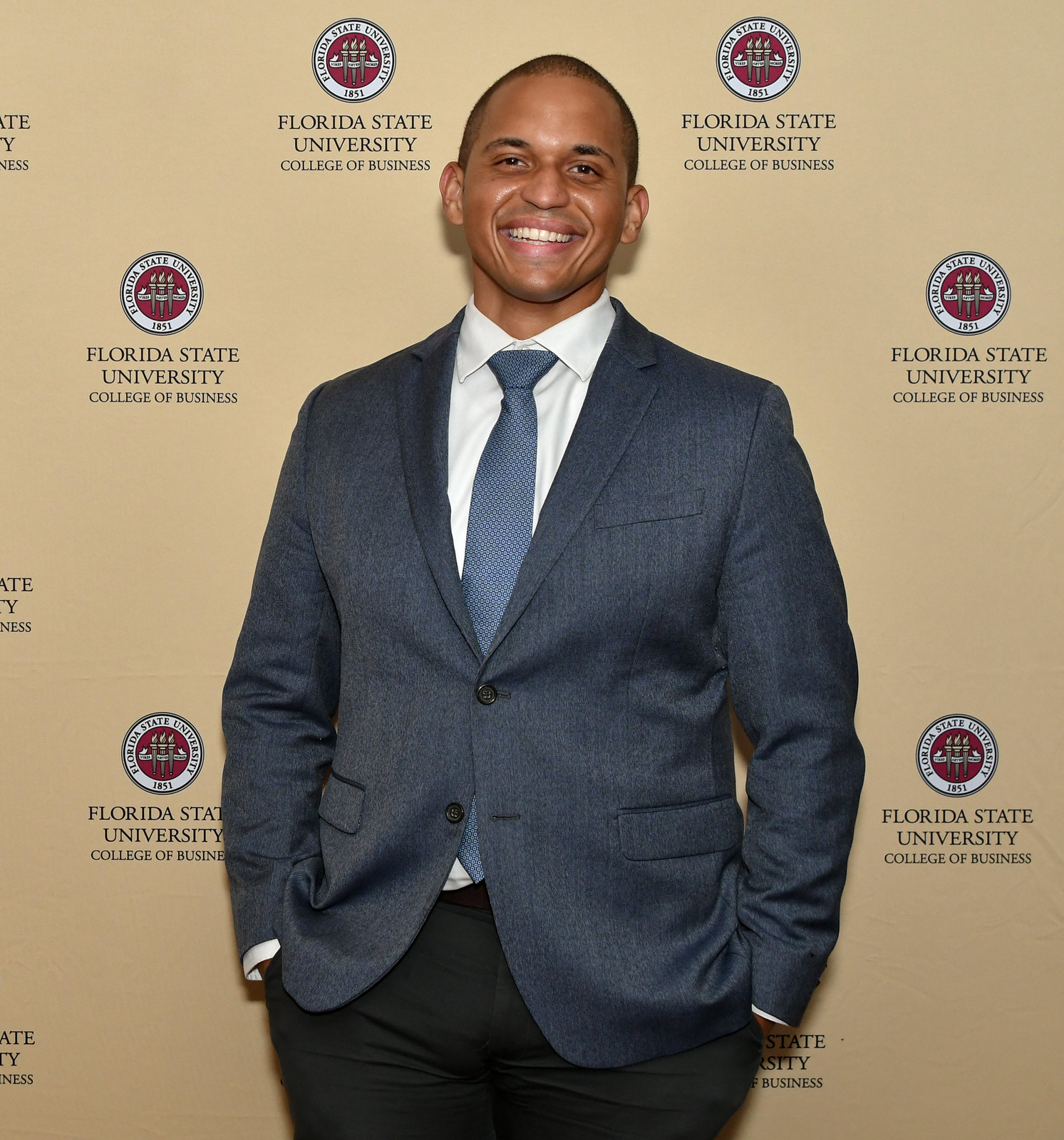In a well-lit area, a smiling African American man in his early 40s, who bears a resemblance to the actor Hill Harper, poses confidently for the camera. He stands against a tan, neutral-colored backdrop adorned with repeating Florida State University logos, each featuring a circular design. The logo consists of an outer white circle reading "Florida State University 1851" and an inner red circle showcasing three flaming torches encircled by a banner. Beneath the logo, "Florida State University College of Business" is inscribed. The man exudes professionalism and warmth, his short, dark hair closely shaved. He is outfitted in a dark blue sport jacket with a single button fastened at the top, paired with dark pants—either black or very dark blue. He wears a crisp white shirt and a blue tie adorned with subtle white dots. His hands rest casually in his pants pockets as he stands poised and approachable.